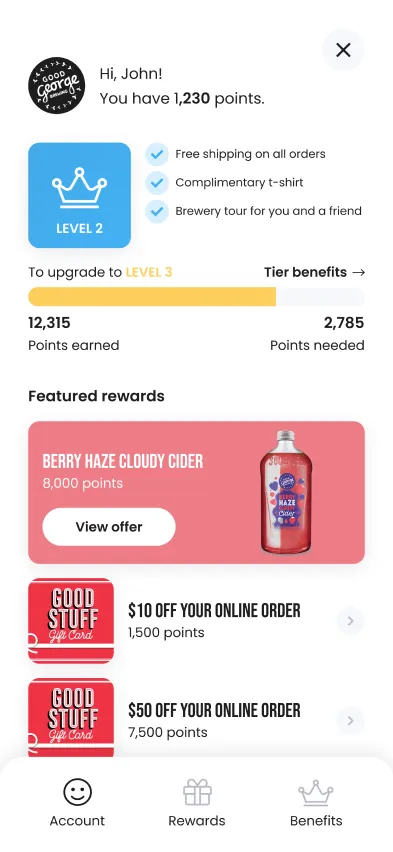The image starts at the top with a greeting text in white font that reads, "Hi, John. You have 1,230 points." To the left of this text, there is a black circle with white font that says, "Good, George."

Below this, there is a blue rectangular box with white font that indicates "Level 2." Inside the box, there is also a white outlined crown symbol.

To the right of the level indication, there are three checkboxes with respective benefits listed:
1. Free shipping on all orders.
2. Complimentary t-shirt.
3. Brewery tour for you and a friend.

Underneath the checkboxes, there is a prompt to "Upgrade to Level 3." It provides the following information:
- Points earned: 12,315
- Points needed: 2,785

At the bottom, the image highlights a section titled "Featured Rewards," followed by an entry for "Barry Hayes Cloudy Cider."